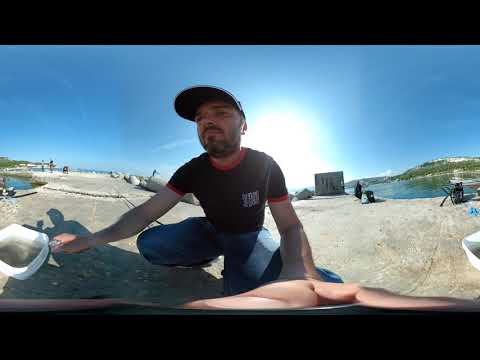The image is a vibrant selfie taken at a scenic lakeside, likely using a selfie stick, which has caused the man's left hand, holding the camera, to appear large and close to the lens. The man is kneeling or squatting, facing the camera, and wearing a black t-shirt with red trim on the sleeves and collar, paired with blue jeans and a forward-facing baseball cap. He sports a relatively new, black beard. In his right hand, he is holding a bucket, possibly for collecting water from the lake. The background showcases a rugged and natural landscape, featuring a dark blue lake or river, a gravelly or sandy shore, hilly terrain with shrubs, and a clear blue sky with the sun shining brightly. The scene also includes people relaxing on what seems to be a concrete pier, typically used for fishing. The wide fisheye lens effect adds a unique, slightly distorted perspective to the photo, highlighting its immersive and casual atmosphere.